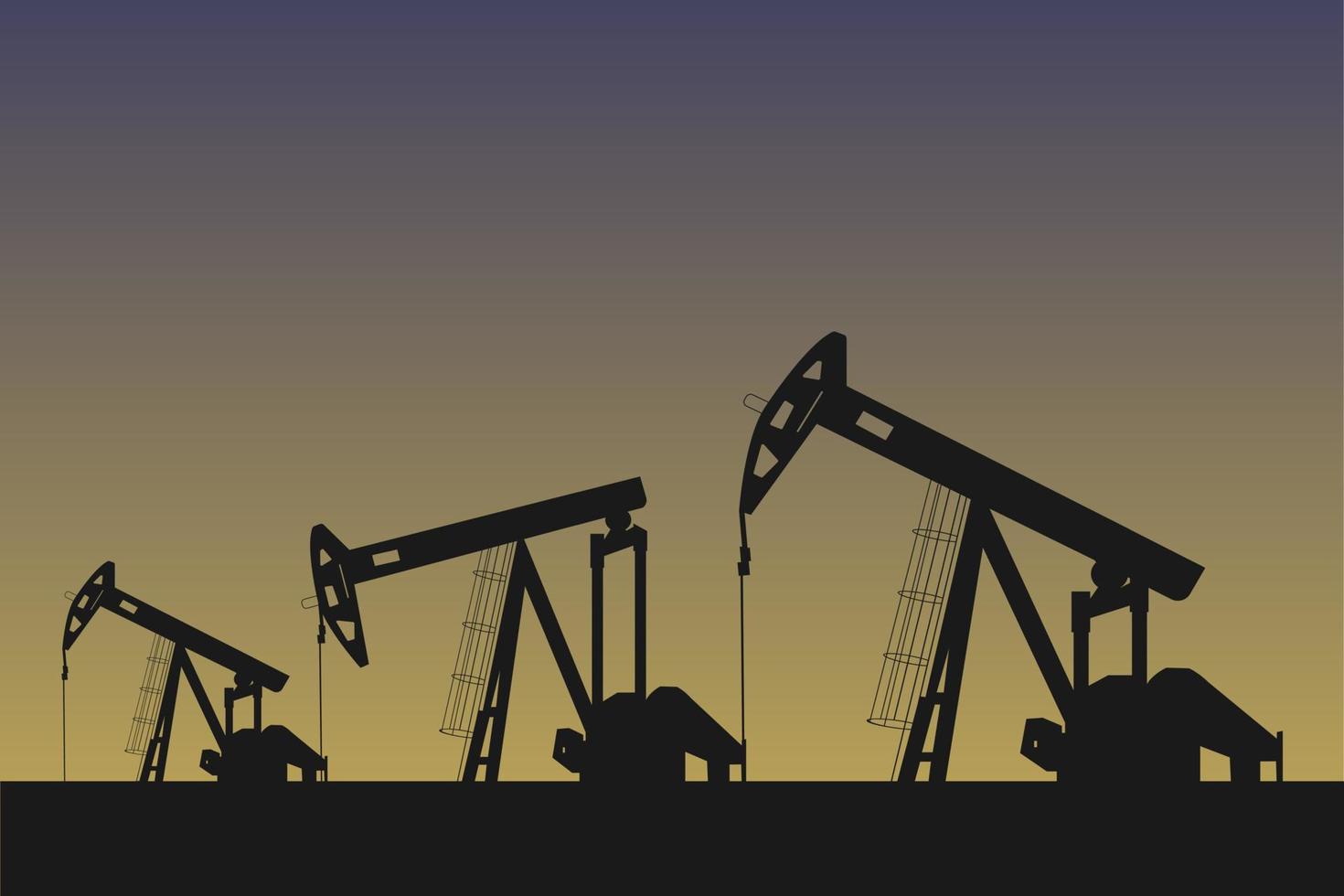This piece of art, resembling a photograph, features a strikingly detailed silhouette of three oil derricks operating at different stages of their pumping cycle. Each derrick, rendered in stark black, contrasts sharply against a softly transitioning background. The gradient begins at ground level with a tan hue, evolving through darker shades of tan and brown, and finally blending into a light gray-purple that deepens to a rich purple at the top, reflecting the dusk sky. The derricks themselves are shown with protective cages for workers and cables extending into the ground, highlighting the industrial activity of oil extraction. The middle derrick is slightly larger, suggesting a depth of field. The composition, devoid of text and minimally suggestive of its location, conveys a moody and stark atmosphere through its robust use of silhouettes and a nuanced color palette in the background.